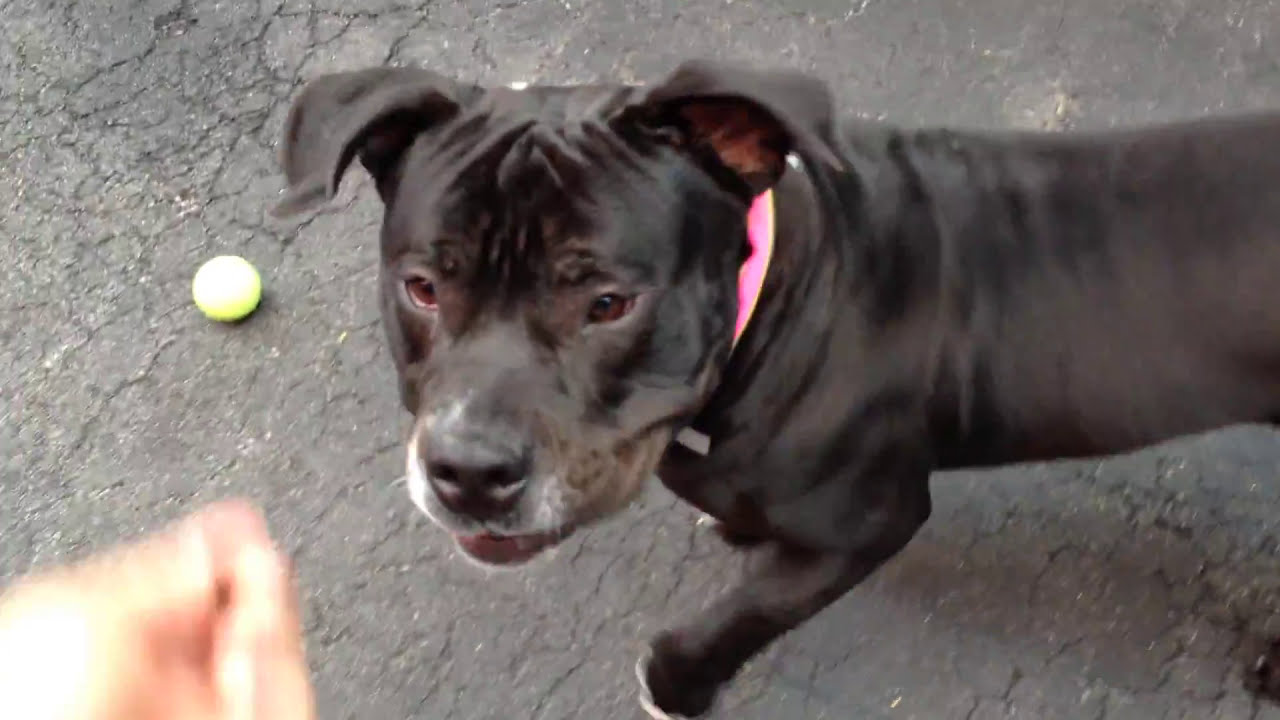In the image, a young black puppy, possibly a pit bull mix, is the central focus. He stands on a cracked, dark asphalt driveway with a visible chip holding a shallow puddle of water. The puppy is adorned with a bright orange-pink collar with a hint of yellow, and you can see a little bit of white peeking out from the bottom of the collar and his nose. His forehead shows prominent wrinkles, giving him an inquisitive expression as his attentive brown eyes and pointy ears with a touch of pink inside focus on a blurred hand in the bottom left corner, seemingly offering him a treat. One of his front paws displays a bit of white, while his body is angled to the left, making his other paws and tail not visible. On the ground beside him lies a small yellow and green ball, suggesting a recent game of fetch. The overall composition of the photo is slightly blurred, emphasizing the interaction between the person and the curious puppy.